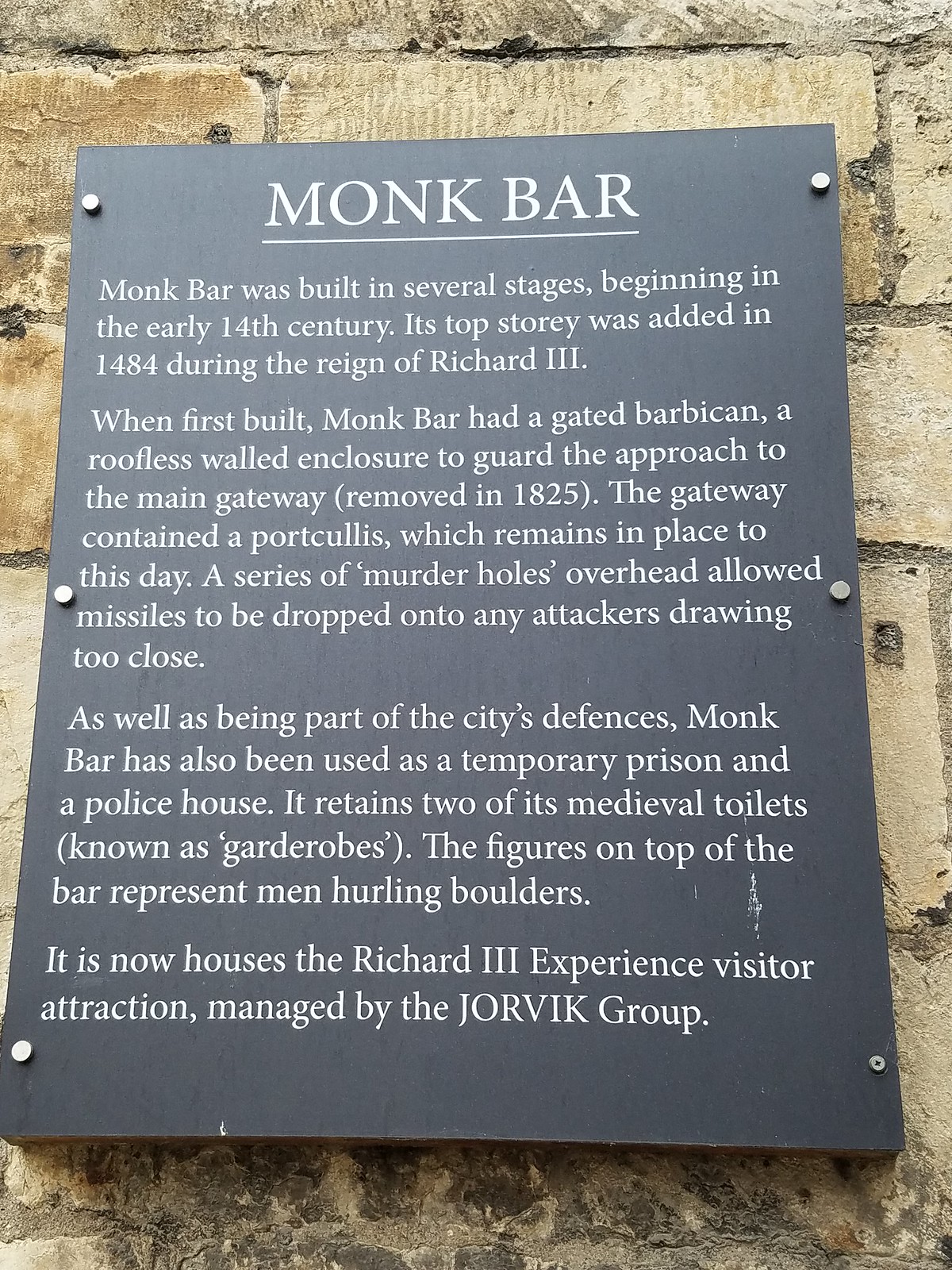This photograph captures a detailed plaque, fastened to a whitish and brownish brick wall, describing the historical Monk Bar. The plaque, made of metal with a black background and white text, provides an informative overview of Monk Bar. At the top of the plaque, the words "Monk Bar" are prominently displayed in all capital letters. Below this heading, the plaque describes the multi-stage construction of Monk Bar, beginning in the early 14th century, with its top story being added in 1484 during the reign of Richard III.

Originally, Monk Bar featured a gated barbican—a roofless walled enclosure designed to protect the main gateway— which was removed in 1825. The gateway still contains a portcullis, and a series of murder holes above allowed defenders to drop missiles onto approaching attackers. Additionally, the plaque mentions Monk Bar's usage as a temporary prison and police house and notes the retention of two medieval toilets, known as garderobers. The figures on top of the bar are described as representing men hurling boulders. Today, Monk Bar houses the Richard III Experience Visitor Attraction, managed by the Jorvik Group.